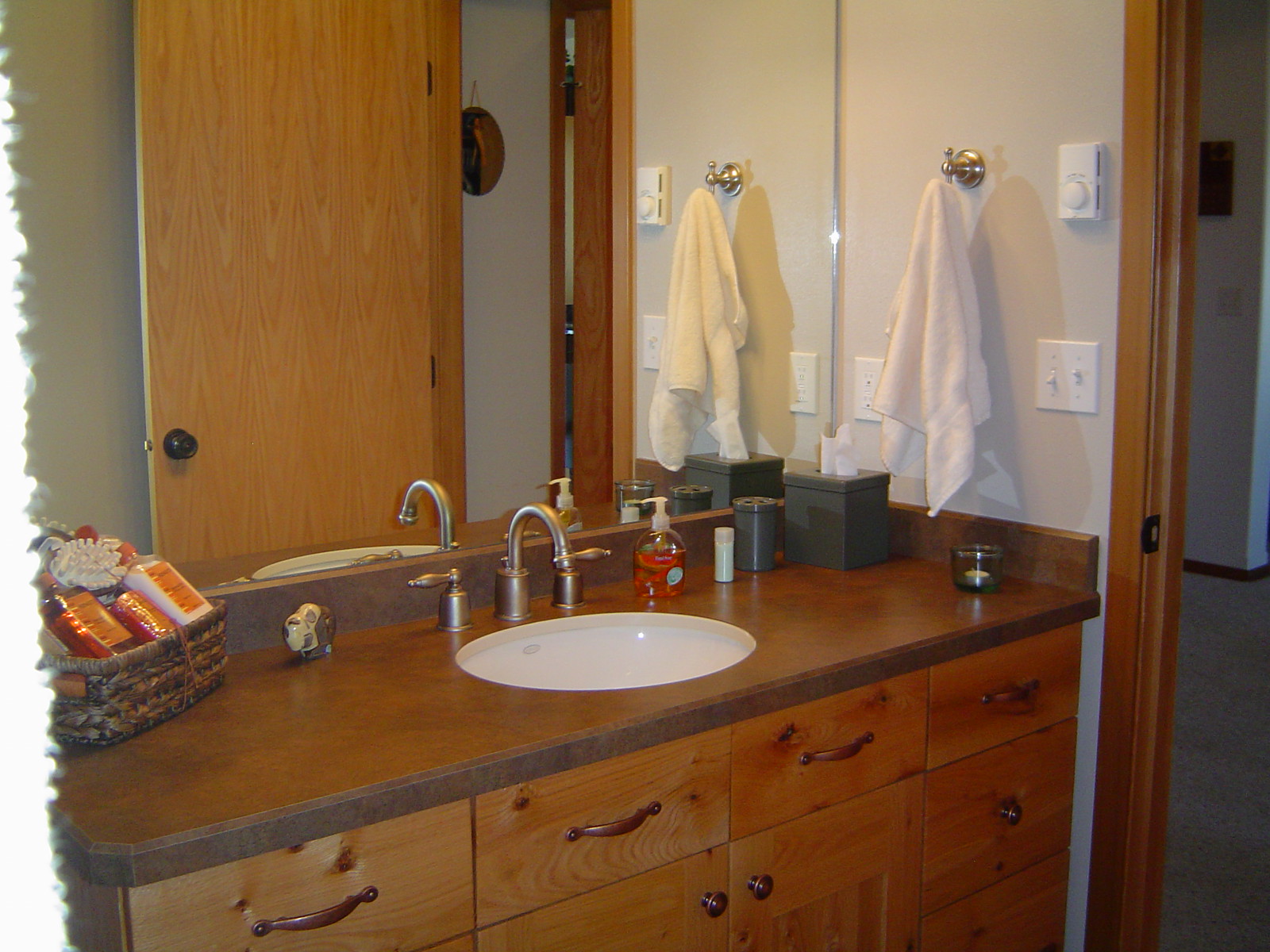In this image of a bathroom, we observe a detailed and intriguing setup. On the right side of the frame, a door with a brown-trimmed frame opens into an adjacent room, revealing a white wall adorned with a black object and a baseboard trimmed in black. The carpet in this adjoining room appears to be a tan or grayish color.

Back in the bathroom, the left side of the image appears faded or ruffled, possibly due to some spill or image distortion. The focal point in the center is a mirror mounted on the wall. Above and to the right, a white wall features a silver towel hanger holding a towel. Below this, we find a white box equipped with a knob or dial and a white light fixture with two light switches.

Dominating the lower part of the bathroom, a set of brown cabinets is topped with a grayish-brown counter. This counter holds several items, including a white sink, silver faucet handles, a tissue holder, candles, and a gift basket containing body wash and cleaning supplies. Furthermore, on the left side of the counter, there's a brown basket.

Reflecting in the mirror, we glimpse a brown door and a round picture hanging on one of the walls, adding to the room’s decorative elements. The detailed arrangement and color coordination give this bathroom a warm and inviting atmosphere.